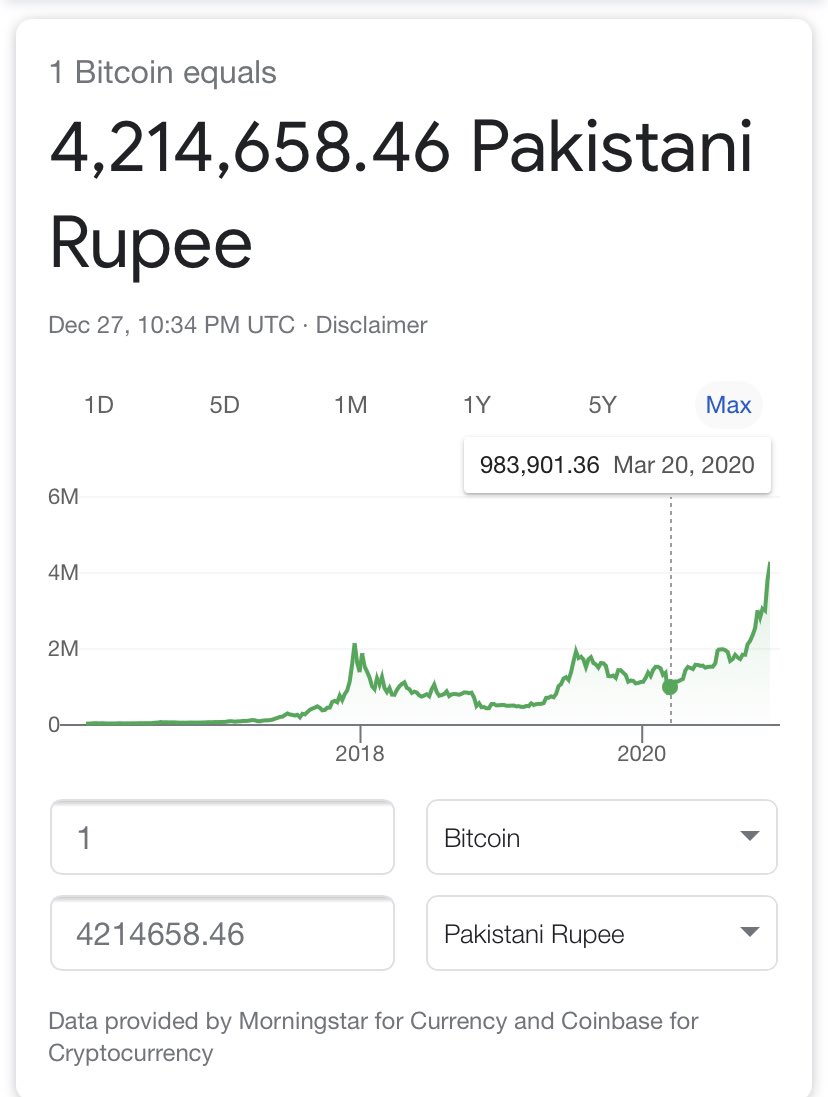This image displays a digital interface for calculating currency exchanges, specifically converting Bitcoin to Pakistani Rupees. At the top, it prominently states: "1 Bitcoin equals 4,214,658.46 Pakistani Rupees," timestamped at 10:34 p.m. UTC on December 27th, though the year is unspecified. 

A clickable "disclaimer" link is seen below this information. Beneath it is a detailed chart, which tracks the historical value of Bitcoin relative to Pakistani Rupees, starting from before 2018 and extending past March 2020. Notably, the chart shows that on March 20, 2020, 1 Bitcoin was valued at 983,901.36 Pakistani Rupees. The trend in the chart indicates a significant rise starting around 2018, followed by fluctuations, and a considerable increase after 2020. The chart's data line is depicted in green.

The interface includes input fields for different currencies and values. In the first field, the number "1" is entered, with "Bitcoin" specified next to it. Directly below this input, the conversion result is displayed: "4,214,658.46 Pakistani Rupees," which can also be selected from a drop-down menu.

At the bottom, it is noted that the data is provided by Morningstar for currency values and Coinbase for cryptocurrency information.